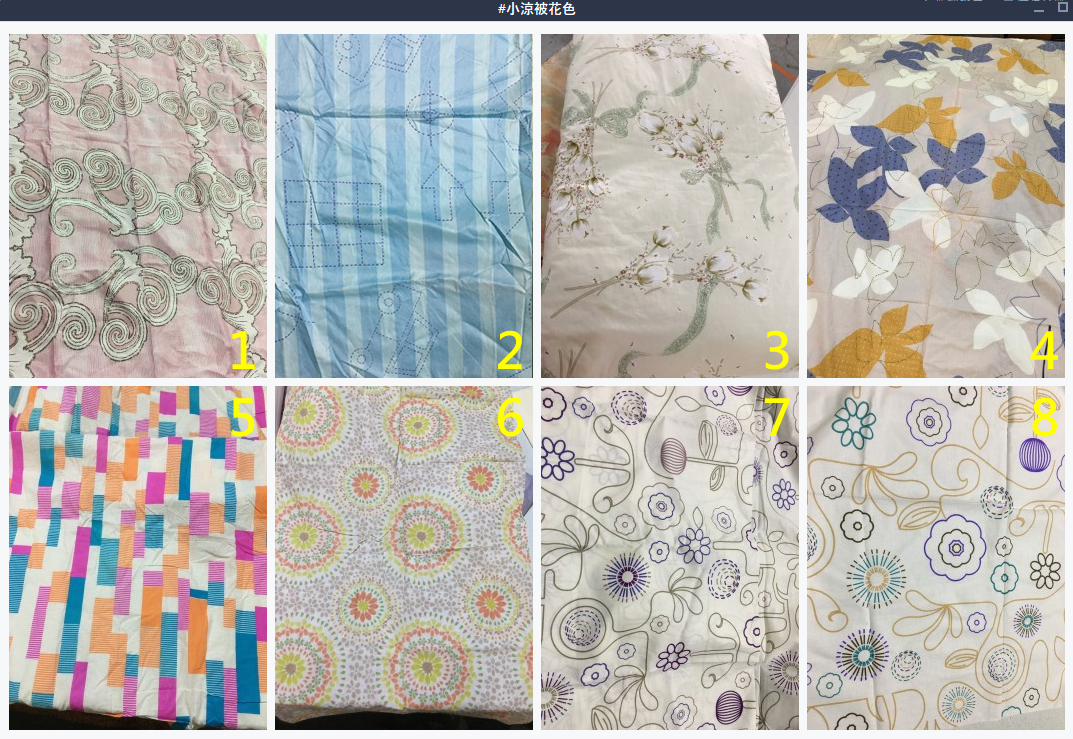This rectangular, horizontal collage image features eight vertically-oriented close-up photographs of various textile patterns, arranged in two rows with four images per row. Each photograph displays a numbered yellow label in the bottom right corner, ranging from 1 to 8. Above the collage, there is Asian writing in white font on a horizontal navy-blue or black strip. 

The first image showcases a light pink fabric with an intricate scrolling white pattern, possibly resembling paisley. The second image displays alternating light blue and medium blue stripes with dotted figures, including a car and some arrows and checkboxes. The third image has a cream background adorned with white flowers, brown accents, and green ribbons. 

The fourth image features a cream-colored fabric with medium blue, orangey-yellow, and white decorations, some of which resemble birds clustered together. The fifth image highlights a white background with vibrant splashes of orange, turquoise blue, and hot pink-purple in abstract, intertwined lines. 

The sixth image is on a cream backdrop with small purple flowers and circular designs, containing orange and green sunflower-like figures. The seventh fabric is an off-white color embellished with black, purple, and gray floral and leaf patterns. Finally, the eighth image, similar to the seventh, includes additional brown and blue-green floral and leaf motifs.